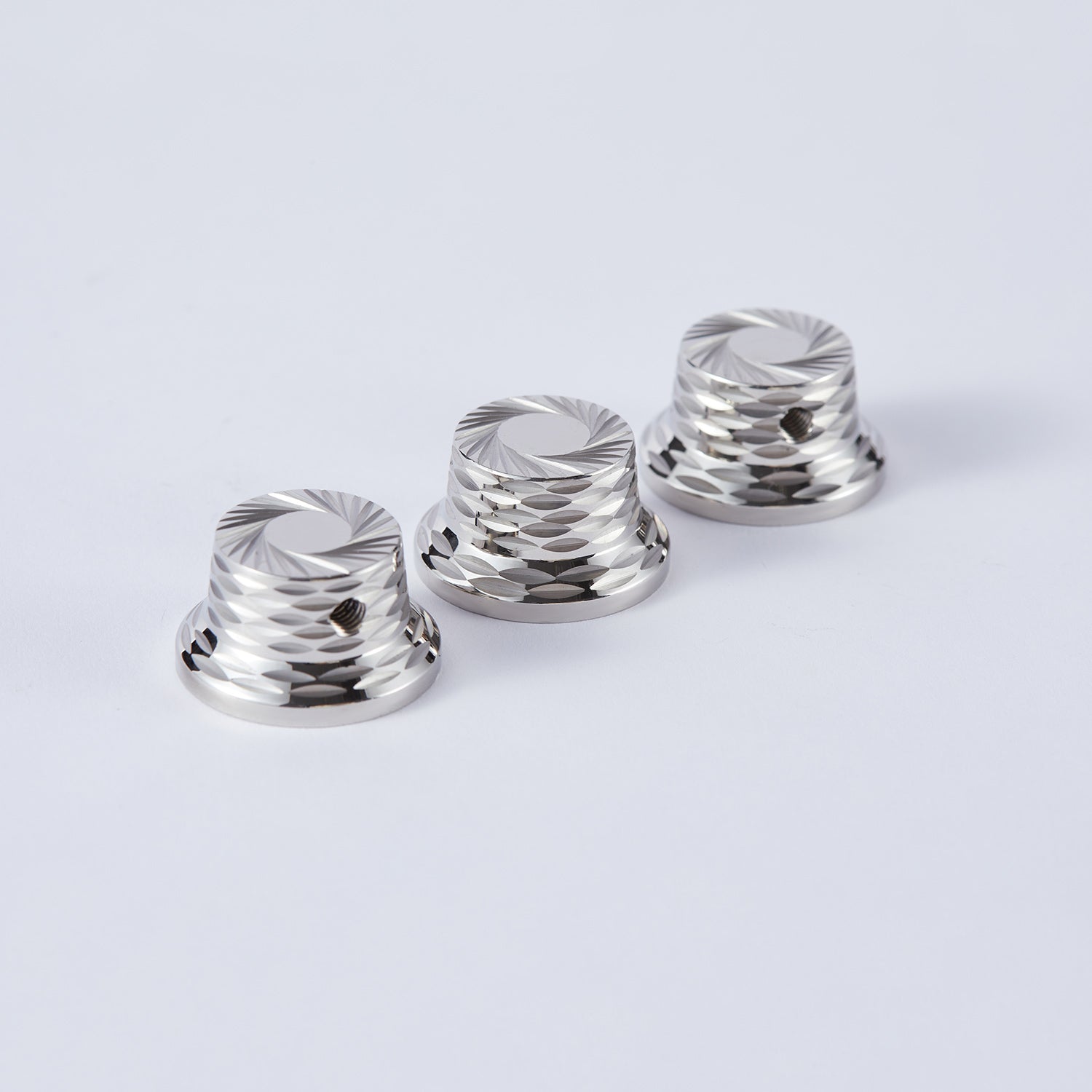The photograph depicts three shiny, cylindrical metal objects, likely knobs, arranged in a diagonal row from the lower left to the upper right corner. The knobs, which appear to be made of chrome or a similarly shiny silver metal, rest on a white surface and cast subtle shadows that emphasize their form. Each knob is wider at the base than at the top, featuring intricate carvings and a spiral pattern on their flat tops. These grooves radiate from a plain central disk out to the edge. Additionally, each knob has a threaded hole on the side, suggesting they are designed to be secured with a set screw, potentially for use on an electric guitar.